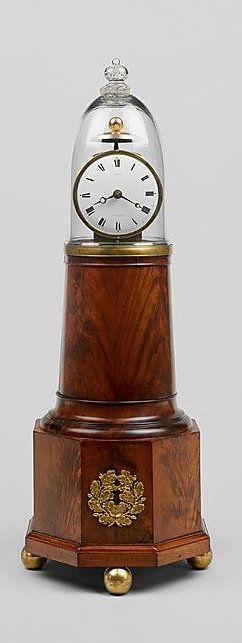The image depicts a tall, narrow pedestal clock, about four times as tall as it is wide, set against a medium gray background. The base of the clock features four gold spherical legs, providing a stable foundation for the intricate wooden pedestal, reminiscent of cherry wood in color. This wooden structure, designed with an octagonal shape at its base, narrows and transitions into a more cylindrical form as it ascends. Near the top, the wood is complemented by a gold band, above which a clear glass dome encloses the clock. The dome encases a white-faced clock with black Roman numerals and hands, and a small gold ornament just below the clock face. The overall design has a lighthouse-like appearance, with detailed craftsmanship accentuating its elegant form. The time reads 8:20.